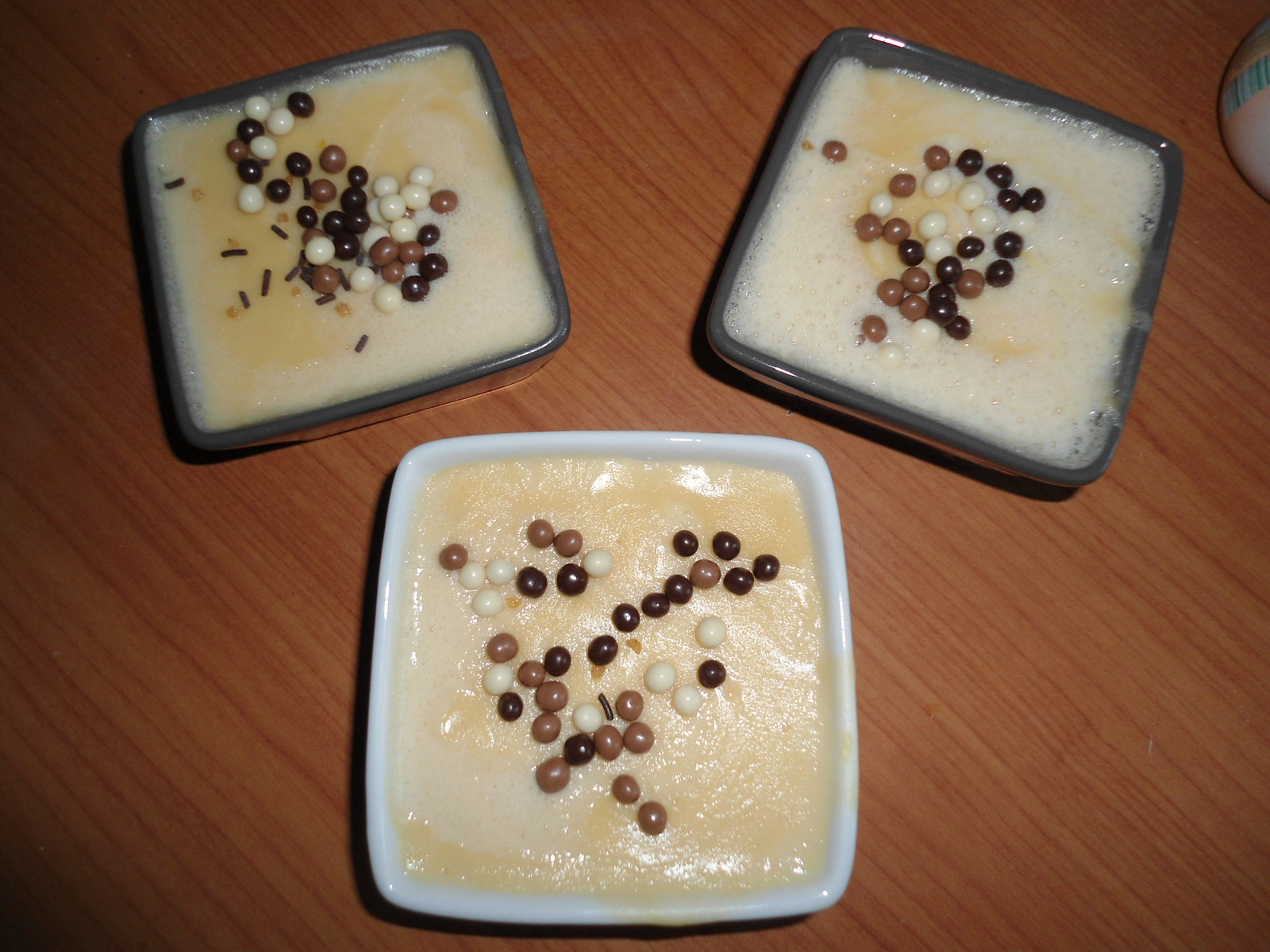This is a top-down image of a tabletop with a faux wood effect, featuring three square ceramic casserole dishes containing a yellowish-white pudding mixture. The table, resembling medium brown wood with an orange tint, appears varnished and new. The front dish is white, while the two in the back are gray. The pudding in each dish is topped with scattered chocolate balls in dark, milk, and white varieties, adding to the texture and color contrast. Harsh overhead lighting creates shadowed edges and reflections on the table. There is a fourth dish slightly encroaching into the top right corner of the image, with unclear details.